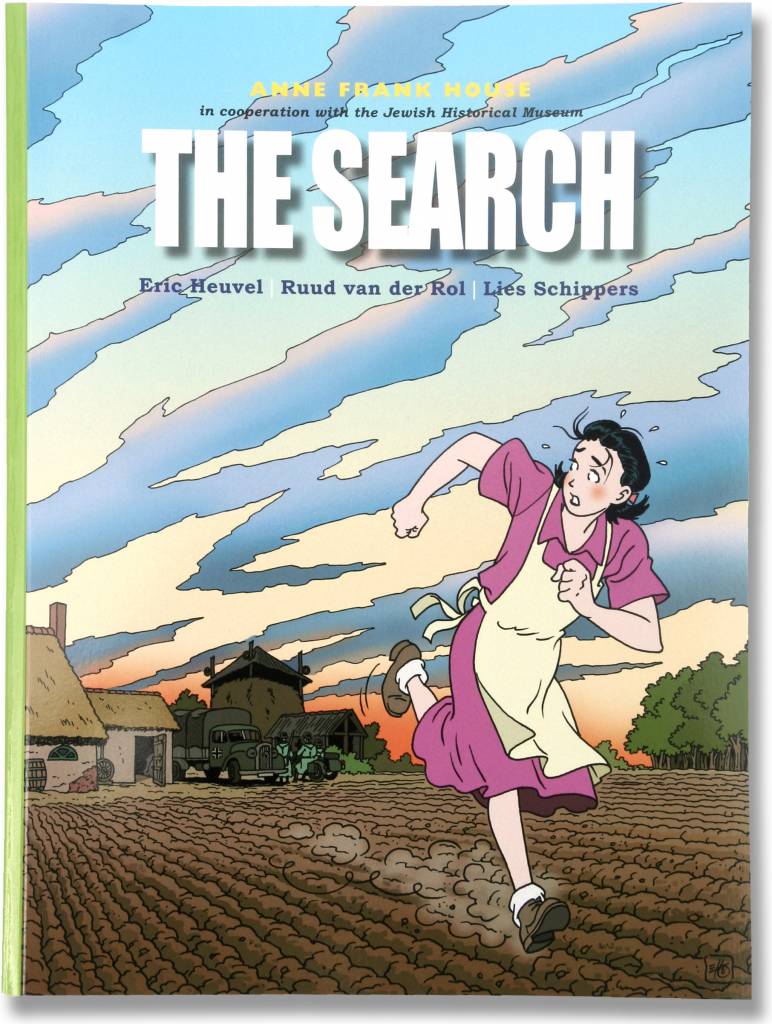The image is a detailed cover of a book titled "The Search." At the top, in a yellow font, it reads "Anne Frank House in cooperation with the Jewish Historical Museum," and just below in large, white capital letters is the book's title. The authors listed beneath are Eric Heuvel, Ruud van der Rol, and Lies Schippers in blue text. The book's spine on the left side is green.

On the cover, a young girl in a pink dress with a white apron is prominently featured. She appears to be running across a barren, farm-like field with brown dirt and sporadic green trees. The girl, who is wearing brown shoes with white socks, looks frightened and is sweating, with visible beads of sweat on her head. In the background, there's an orange-hued sky that transitions to blue with jagged gray clouds. Far off in the distance, a green truck is parked near a couple of brown buildings, likely a farmhouse. The overall scene suggests a tense and urgent atmosphere.